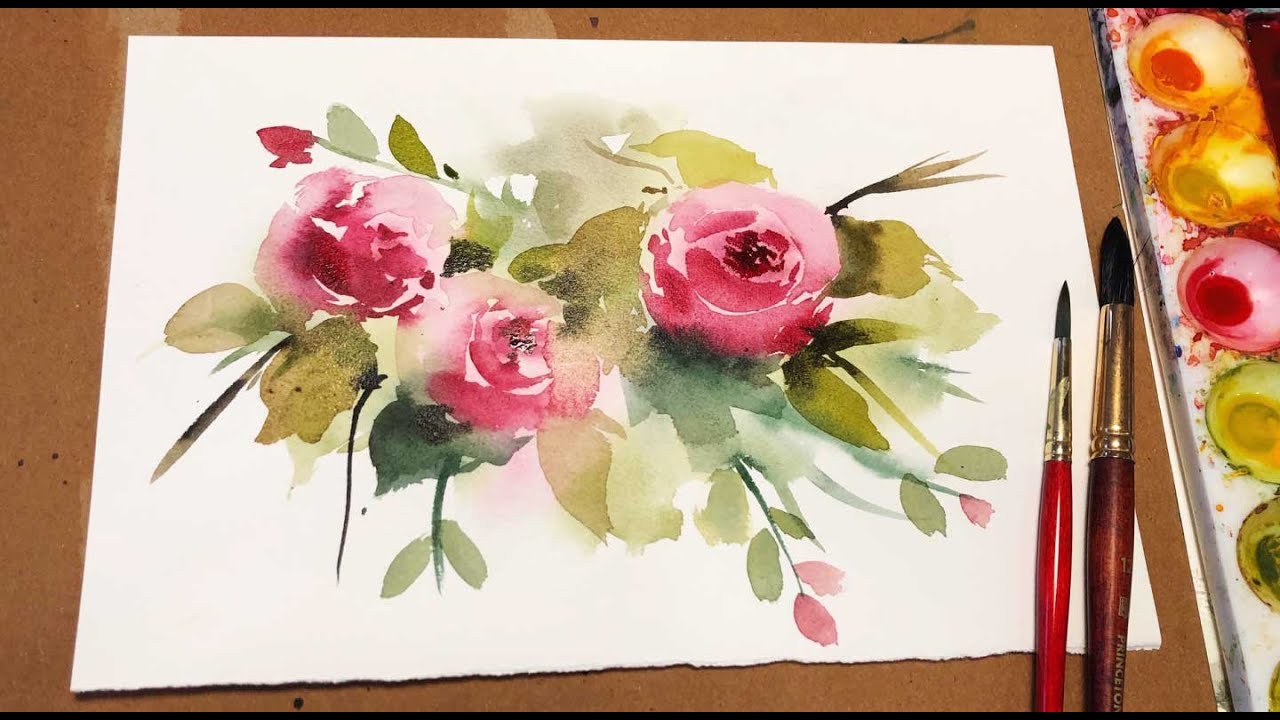The image depicts a detailed and vibrant watercolor painting of three blooming roses on a piece of white parchment, which is set against a dark brown wooden drawing board. The roses are painted in a striking pinkish-red hue with deep red contours and delicate white highlights, surrounded by pale green leaves rendered in the soft, blotchy style characteristic of watercolor. The artwork, which appears to be a work in progress or just completed due to the absence of a signature, includes two paintbrushes with different-sized tips; one has a red handle, and the other has a brown handle. These brushes rest on the lower right corner of the parchment. Adjacent to the brushes, there is a white plastic watercolor palette featuring five concave wells containing various colors: an orangish-red, an orangish-yellow or gold, a pink, an avocado green, and a darker green partially cut off by the edge of the drawing board. The entire setup suggests a dedicated and ongoing artistic effort.